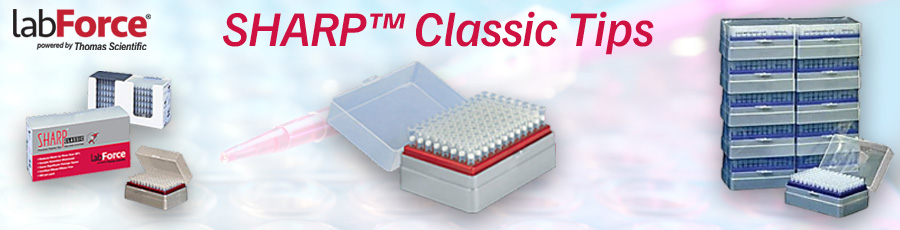The image showcases an advertisement for medical supplies. In the upper left corner, a black and red label prominently displays "Lab Force," followed by black text beneath reading "powered by Thomas Scientific." Below this, there are several boxes: a mixture of white, red, and gray boxes, with one in red text reading "Sharp™ Classic Tips." Centrally, there is a gray box with a red inset, filled entirely with numerous small white-tipped micro-pipette vials. To the right, a similar display shows additional boxes, this time with blue insets—each also containing white-tipped vials. The overall design hints at an old-fashioned aesthetic, emphasizing the product, "Sharp Classic Tips," seemingly for the purpose of lab work, although their exact application remains unidentified.